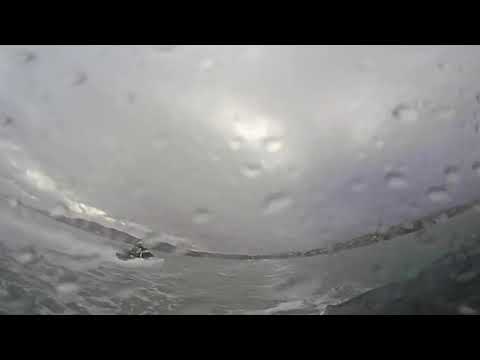The photograph captures a somber, heavily clouded scene where the sky is predominantly gray, suggesting an impending rainstorm. The image is taken with a lens covered in numerous transparent water droplets, which distort and obscure the clarity. The body of water occupies the bottom portion of the image, arching in a graceful U-shape from right to left. The water, characterized by its blue-gray tint and occasional white patches of foam, appears to be either a river or sea.

In the center-left of the image, partially shrouded by the water droplets, there is a small, black vehicle—likely a jet ski or boat—trailing white foam from its sides and behind, suggesting motion. The rider, dressed in all black and gray, adds to the overall monochromatic theme. The distant background reveals low-lying hills or rocks, adding depth and context to the landscape. The upper part of the photograph features a dark gray sky with patches of white clouds and a hint of blue to the right, and two black bars frame the top and bottom of the image. The lens's water droplets and the grayscale palette combine to convey a moody, atmospheric scene.